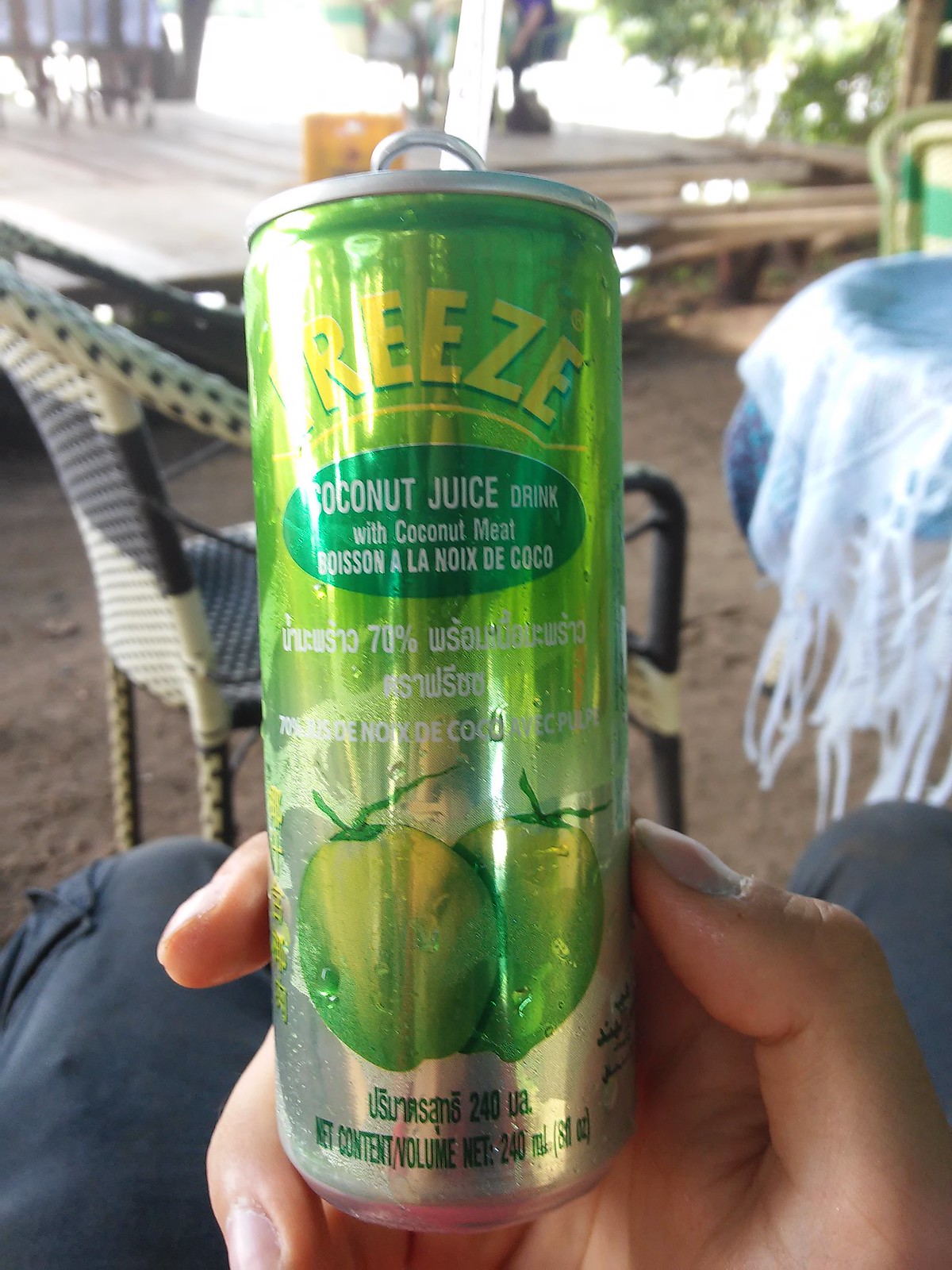This image captures a close-up of a hand holding a lime green can of coconut juice drink branded as either "Breeze" or "Freeze," although the first letter is obscured by a glare. The can is slender and has a silver rim with yellow lettering at the top spelling "Freeze." It features a dark green circle with the text "coconut juice drink with coconut meat" and an illustration of two young green coconuts. Near the bottom, in green text, it states the net content volume of 240 milliliters (8 fluid ounces). The person holding the can is wearing blue pants, and the can is grasped with their right hand, the thumb on the side and the middle finger supporting the base.

The scene appears to be outdoors on a patio area, with a sandy beach visible in the background. There's a brown and white chair to the left and a blue-covered table to the right. The overall setting exudes a relaxed, beachside ambiance, with additional tables and chairs scattered around, suggesting a leisurely, tropical environment.